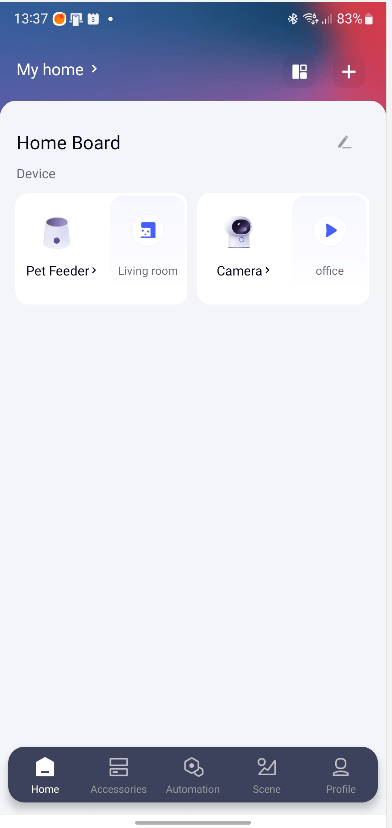This image depicts a screenshot of a mobile device, potentially a phone or tablet, as evidenced by the status bar at the top of the screen. The time displayed is 13:37 and various icons are visible, including indicators for Bluetooth, Wi-Fi, and a battery level at 83%. 

At the top of the page, there is a home button on the left and an icon resembling a grid of squares on the right, which possibly opens another home screen. Adjacent to the grid icon is a plus icon, which might be used to open or add new elements to the home screen.

Below the status icons, there's a section labeled "Home Board" with an adjacent edit icon. Below this, the screen displays categories such as "Device," "Pet Feeder," "Living Room," "Camera," and "Office."

Further down, the interface includes navigation buttons labeled "Home," "Accessories," "Automation," "Scene," and "Profile." The overall design utilizes a gray and white color scheme, accented with a blue and red top border. The bottom navigation row is in a dark navy blue color.

The layout and elements suggest the interface might be from a smart home monitoring or management application.